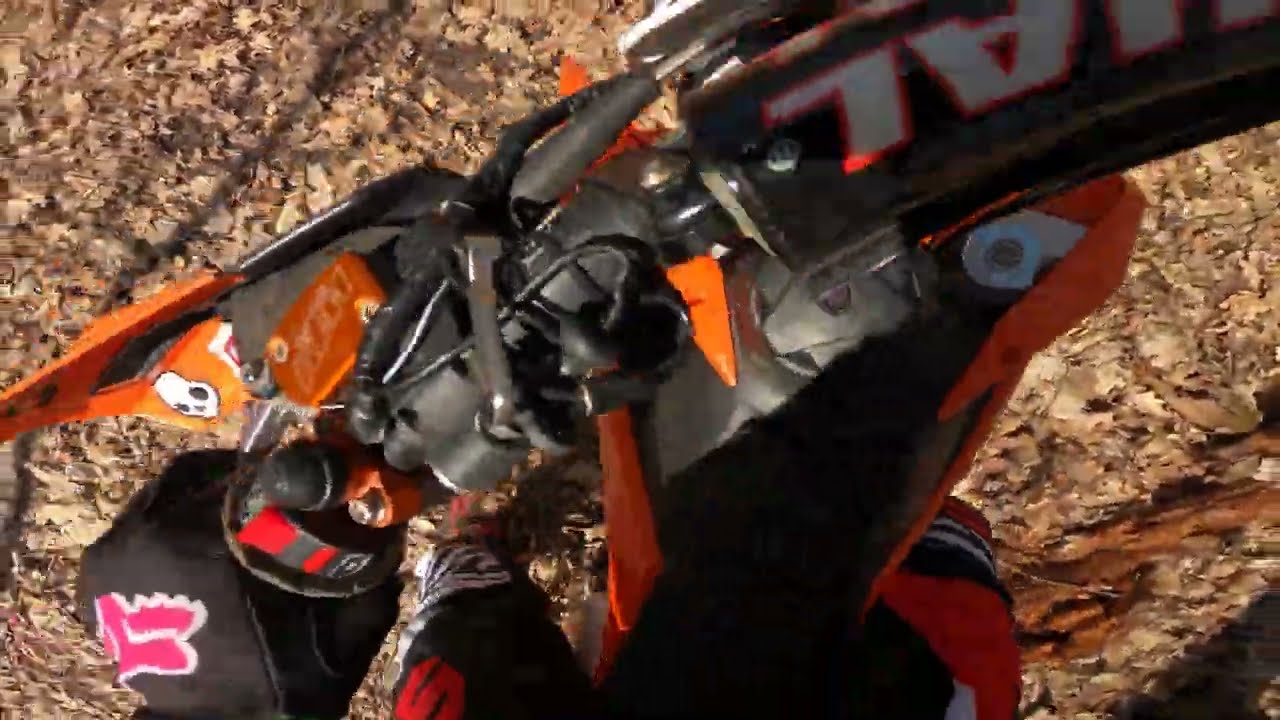The image shows a mechanical or possibly tool-like object resting on a bed of scattered brown leaves, likely indicating an autumn setting. The object predominantly features black and metallic parts with orange accents and appears complex, with components resembling levers, gears, and hoses. The central portion of the image includes a visible orange rectangle, possibly a reflector, and there are letters, particularly "A" and "L," in upside-down white font outlined in orange, hinting at some form of branding or labeling, although the full text is cut off. A black bag with a pink figure or logo, featuring unreadable but heavily outlined text, is situated on the lower left side of the image. The background comprises numerous autumn-colored leaves, giving a natural, earthy tone to the scene. The ambiguity of the object's function suggests it could be a motorcycle part, a weapon, or some intricate piece of machinery, heightening the mysterious and technical feel of the photograph.